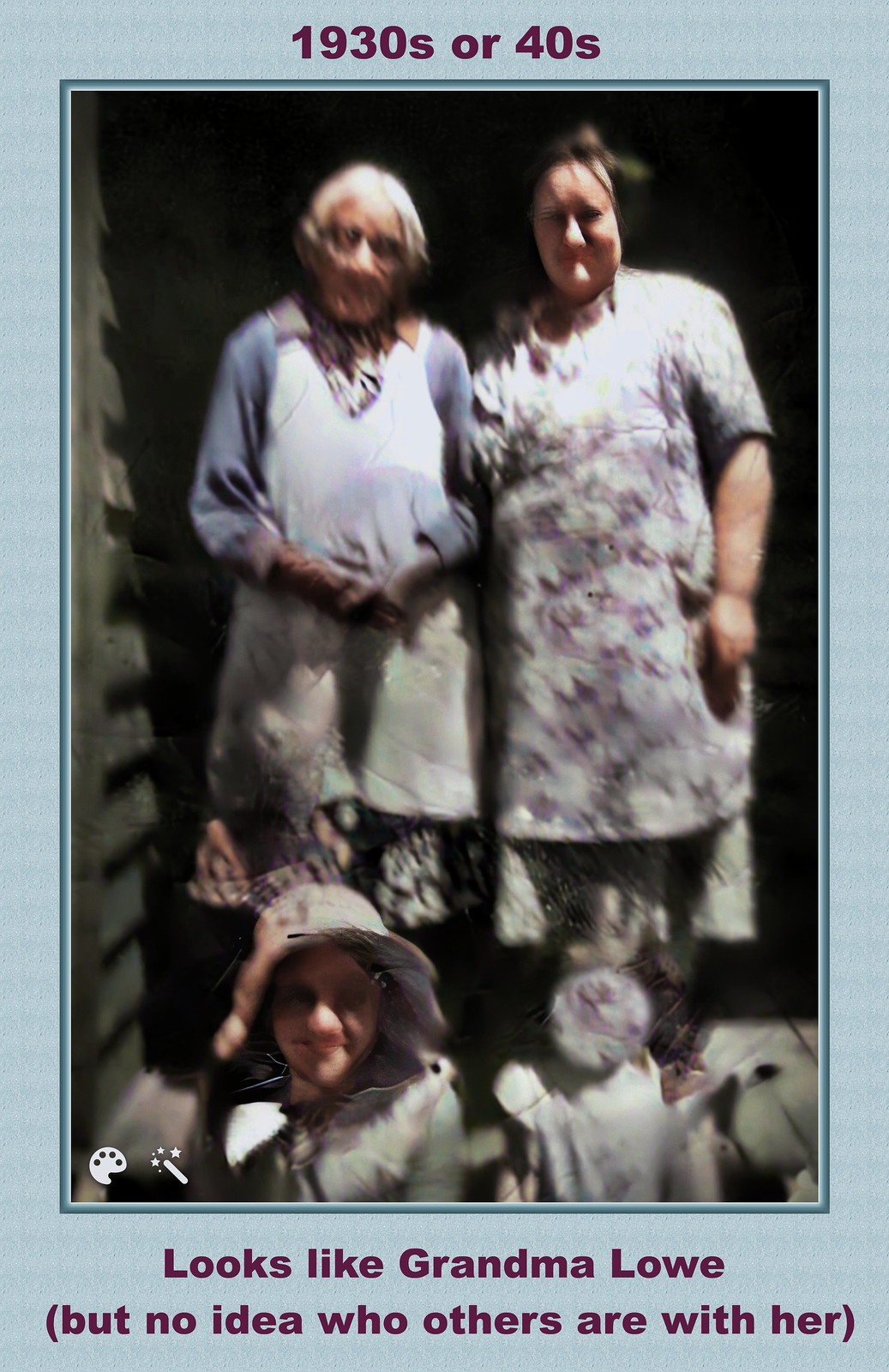This portrait-oriented photograph, framed in a light blue border with "1930s or 40s" written above it in black or possibly red lettering, depicts a scene likely from the 1930s or 1940s. The centerpiece of the image shows two women standing side by side on what appears to be a wooden clap house porch. The woman on the left is quite elderly, seemingly in her 80s, with white hair and wearing a white and blue dress adorned with flowers. Her hands rest in front of her body. To her right stands a younger woman, probably in her 40s, with dark hair. She is dressed in a floral dress and has her right arm placed gently on the back of the older woman. Below them, sitting on the porch steps, are two young girls. The girl on the left, around eight years old, wears a bonnet, while the girl on the right, approximately four years old, is partly obscured by sunlight and possibly a defect in the photograph, making her features difficult to discern. The bottom of the photo reads, "Looks like Grandma Lowe," with a parenthetical note stating, "but no idea who others are with her."